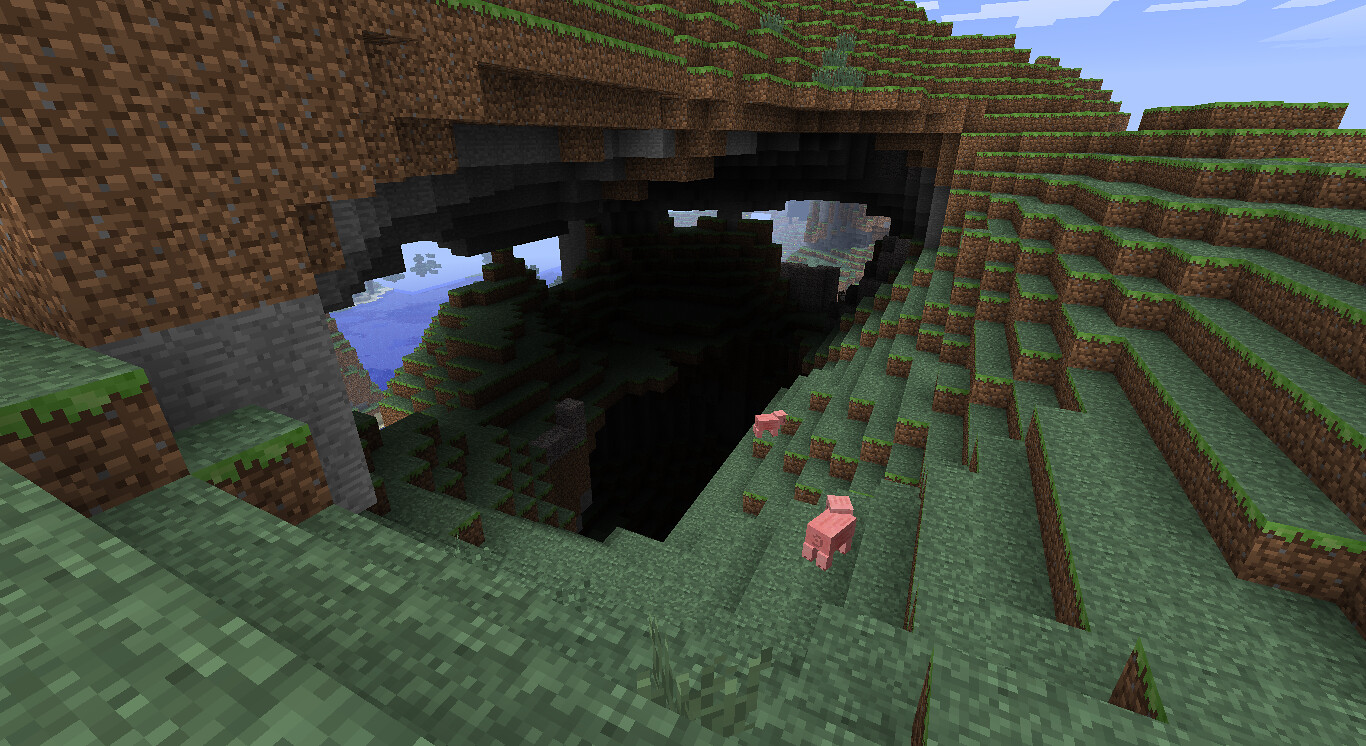This colorful image resembles a scene from a video game, showcasing a blocky, pixelated art style. The central focus is a hill or cliff with a large cave, through which the sea is visible. In the upper right corner, the sky peeks through, adding depth to the scene. The cliff and surrounding ground are composed of blocky textures, with the area beneath the cave resembling a stadium with tiered steps. These steps ascend on the right side and curve around, enhancing the geometric aesthetic. In the middle of this blocky arrangement, there are two squarish, red objects. One resembles a chair, while the nature of the other object remains unclear. The overall composition is decidedly unrealistic, emphasizing the distinctive, cubic nature of the landscape and objects within it.